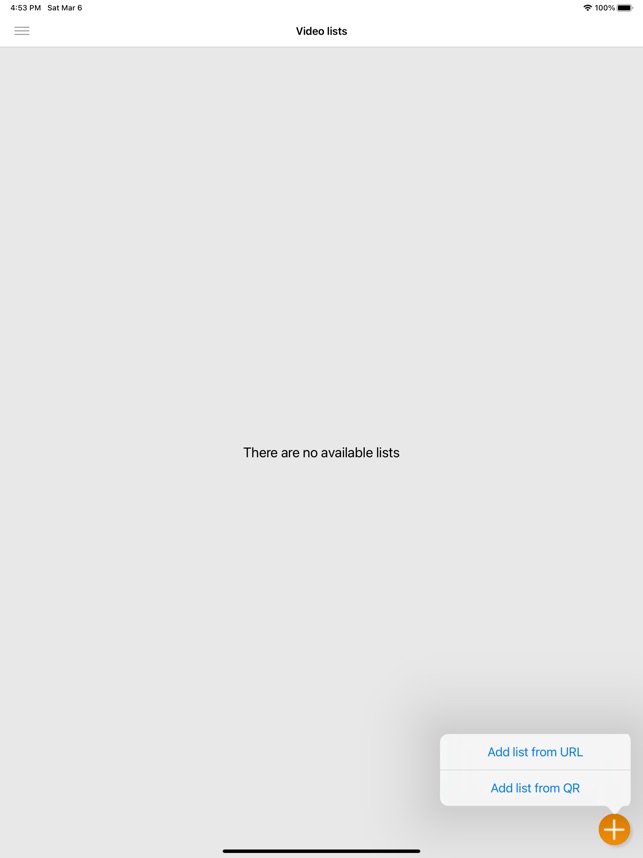This screenshot captures the interface of an iPad app labeled "Video Lists." The title "Video Lists" is centered at the top in small black letters. On the far left side of the screen, a menu icon is visible. The background is a neutral gray, conveying a minimalist design. In the center of the screen, small black print indicates, "There are no available lists," emphasizing the emptiness of the page.

At the bottom right corner of the screen, there's an orange circle featuring a white plus sign. This icon has been activated, triggering a small pop-up box that presents two options: "Add List from URL" and "Add List from QR," both in blue, resembling hyperlinked text. These options suggest the functionality to add video lists from different sources.

Additionally, at the very top right corner of the screen, the status bar displays the time, date, Wi-Fi signal strength, battery percentage, and battery icon, typical of an iPad interface. The overall screenshot provides a clear view of the app's basic layout and functionality options while also capturing the iPad's system details.